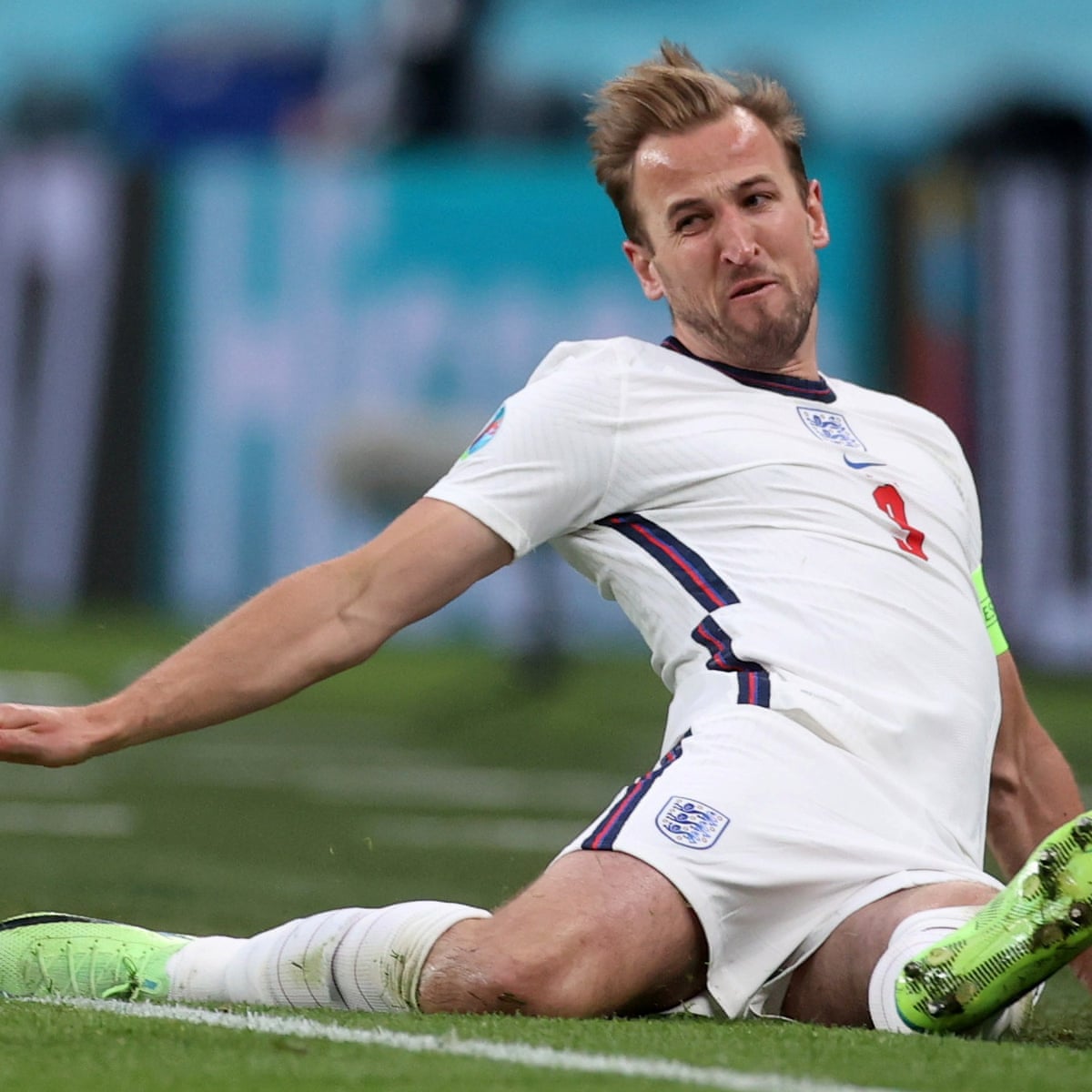This color photograph captures a dramatic moment on the soccer field, featuring a blonde-haired player with spiky hair and a slight beard who has fallen to the ground, performing an unintended splits maneuver. His white uniform, adorned with navy and red stripes along the sides, bears a blue Nike check on the chest and a small, shield-shaped team emblem on one of his short pant legs. Bright mint green cleats and white knee-high socks complete his gear. The athlete's face shows a grimace of pain, suggesting discomfort from the awkward position. The grass beneath him is vividly green, and the background, though blurry, hints at various advertisements set against a light blue backdrop. Despite the blur, the energetic tension of the scene is palpable.